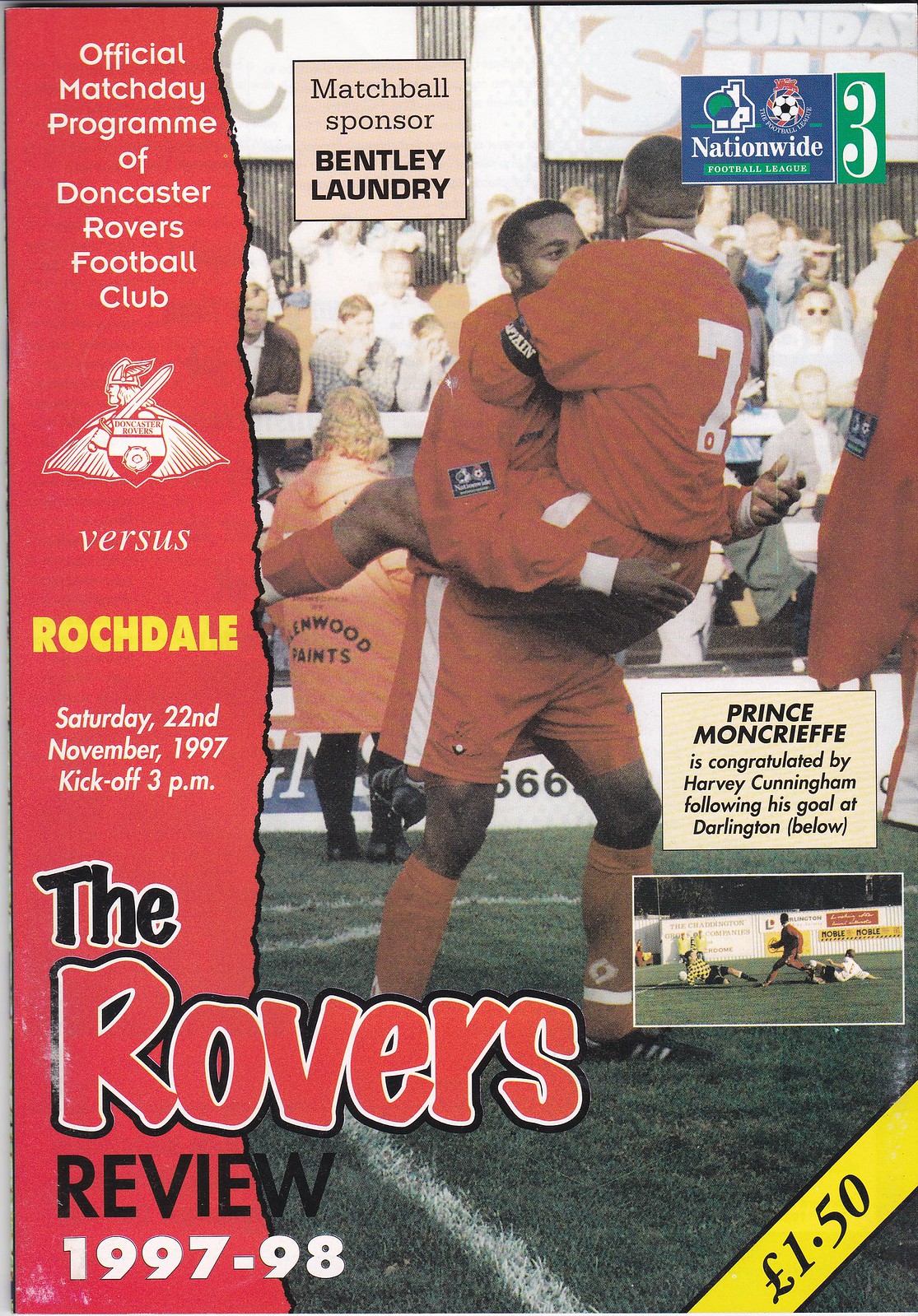This magazine cover, titled "The Rovers Review 1997-1998," features a jubilant moment between two soccer players, both African American, clad in red uniforms. On the field, one player, identifiable by the number seven on his back, leaps into the arms of the other, marking a celebratory moment captured in the image. Surrounding them, additional players and onlookers populate the green field, bordered by stadium stands filled with spectators. Notably, a woman in a long orange coat faces away from the action.

Text elements are prominently featured: a stylized red banner along the left side reads "Official Match Day Program of Doncaster Rovers Football Club," and a logo of a man with a sword is displayed. The opponent, "Rochdale," is highlighted in yellow text, with details of the match scheduled for Saturday, November 22, 1997, at 3 PM. At the bottom left, the series title "The Rovers Review 1997-1998" is present, while the bottom right corner carries a yellow stripe indicating the price of £1.50. Below the main image, the caption notes, "Matchball Sponsor Bentley Laundry. Prince Moncrieff is congratulated by Harvey Cunningham following his goal at Darlington," providing context to the celebratory scene depicted.